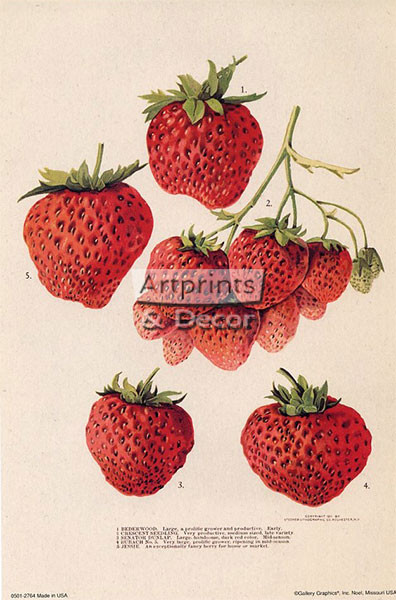This hand-colored poster features the text "Art Prints and Decor" prominently displayed in the center against a light white background. The centerpiece of the image is a detailed cluster of strawberries, predominantly red with visible seeds and green leaves. This cluster is positioned centrally, with the stems and leaves branching off. On the right side of the cluster, there are two unripe green strawberries. Scattered around the central bunch are additional strawberries; one prominent strawberry is located above the cluster in the upper middle, with another to the upper left and two more towards the bottom. Below this central group of strawberries, there is a small paragraph of text rendered in black against the light background, although the text is too small to read clearly. Additional small, unreadable text also appears in the lower left and right corners of the poster.